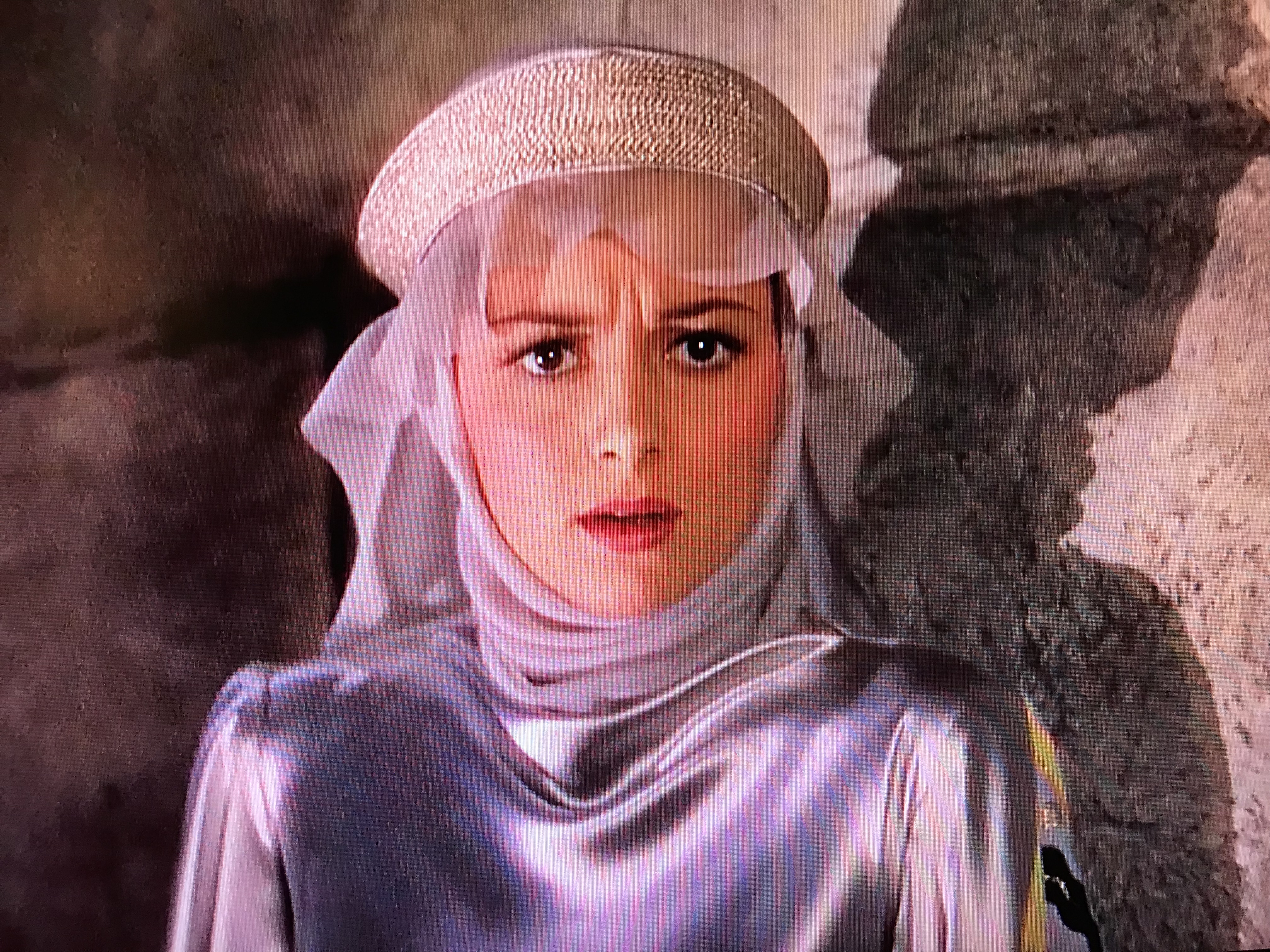The image captures a close-up shot of a woman resembling a character from a video game or an older film, exuding a sci-fi or fantasy vibe. The young lady is adorned in a striking ensemble featuring a silky, shiny silver gown that transitions into a neon purple hue with delicate red and blue accents extending from the chest outward. Her head is encased in a light purple scarf, complemented by a gold headband and a weaved tan hat with frilly details around its edge. She wears red lipstick and blush, with well-defined eyeliner and drawn-on eyebrows, giving her a subtly sophisticated air. Her expression is one of concern or confusion, marked by slight wrinkles between her brows, and her wide, dark eyes reflect a sense of worry. The background reveals an old, cavernous or dungeon-like setting, with grey stone walls flanking either side, adding to the scene's mysterious and atmospheric tone.